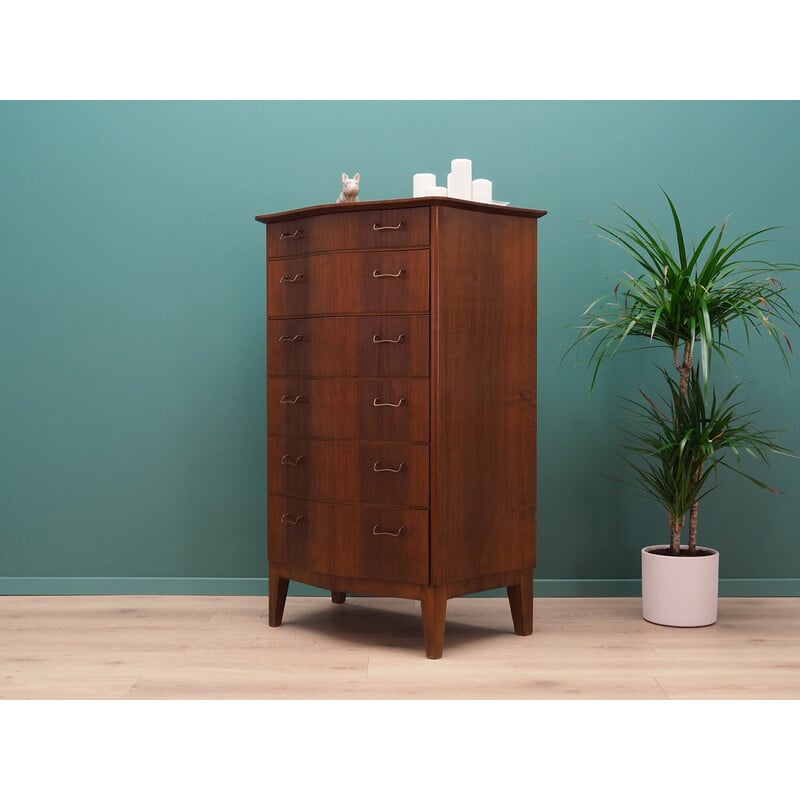This is a detailed photograph capturing the interior of a room. Central to the image is a large, medium dark brown wooden dresser with a visible wood grain, slightly angled away from a greenish-blue wall. The dresser stands on four short legs, elevating it slightly above a light wood or laminate floor with a faint peach tinge. The dresser features six drawers, each with two widely spaced handles. The top drawer is notably shallower, the bottom drawer is the deepest, and the middle four drawers are uniform in size. On top of the dresser sits a small porcelain figurine of a dog and a tray with several white candles of varying heights. To the right of the dresser is a white pot containing three palm trees—one tall and two shorter ones. The wall behind the dresser is greenish-blue with a narrow baseboard, adding a touch of contrast to the scene.